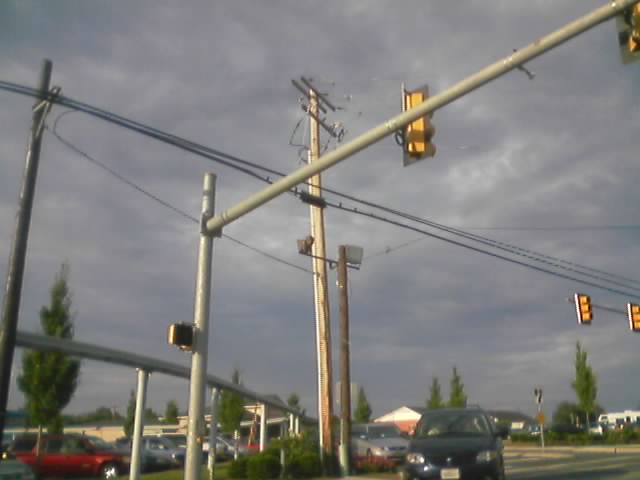In this rectangular photograph, we observe a striking outdoor scene captured during daytime. The sky, which occupies about four-fifths of the image from top to bottom, is a menacing dark gray, suggesting an impending storm. Despite this, there is no evidence of rain as the ground appears dry. Dominating the upper left corner and stretching toward the midsection on the right side, a long telephone wire is suspended above the scene. Below this wire, we find a telephone pole and a streetlight mounted on a silver pole. Beneath the streetlight, several cars are visible, including a prominent black vehicle facing outward on the road. Additional parked cars can be seen in the lower left corner of the image, completing the urban landscape.